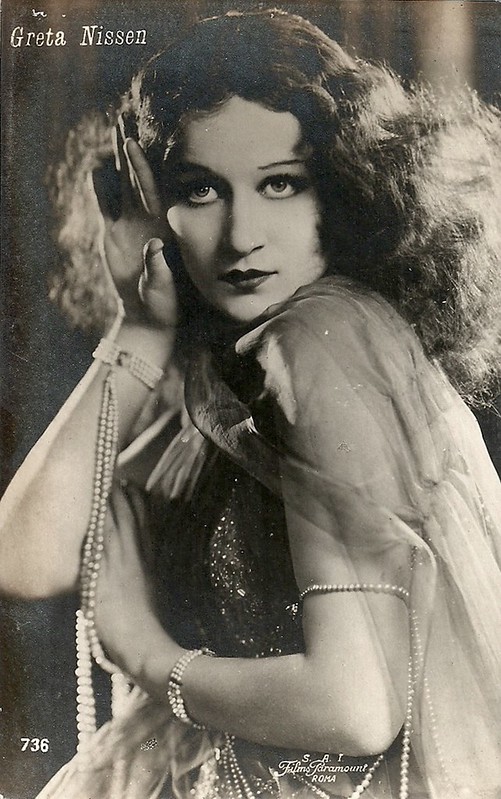This vintage black-and-white photograph features Greta Nissen, a prominent movie star from the early 20th century. Her name, spelled N-I-S-S-E-N, is displayed in white text in the upper left corner, while the bottom corner of the image includes the numbers 736, and words like "Films Paramount" and "Roma." Greta is captured in a glamorous and dramatic pose with her right hand resting against the side of her face. She sports wavy hair that frames her head before cascading past her shoulders, accentuating her expressive eyes, which are emphasized by makeup. Her distinctive, Cupid’s bow lips, likely painted in a vivid red though unseen here in black-and-white, add to her allure. 

Greta is adorned with multiple strings of pearls, one wrapped around her arm and another hanging elegantly down, hinting at her upper-society status or her role as a highly regarded actress or model. Her attire includes a sheer, sparkly gown that reaches down her back, paired with a see-through shawl, allowing a glimpse of her sophisticated yet sensual ensemble. The photograph, marked with texts suggesting it’s a property of a production company, captures her poised in a manner that signifies her importance in the realm of 1920s cinema.